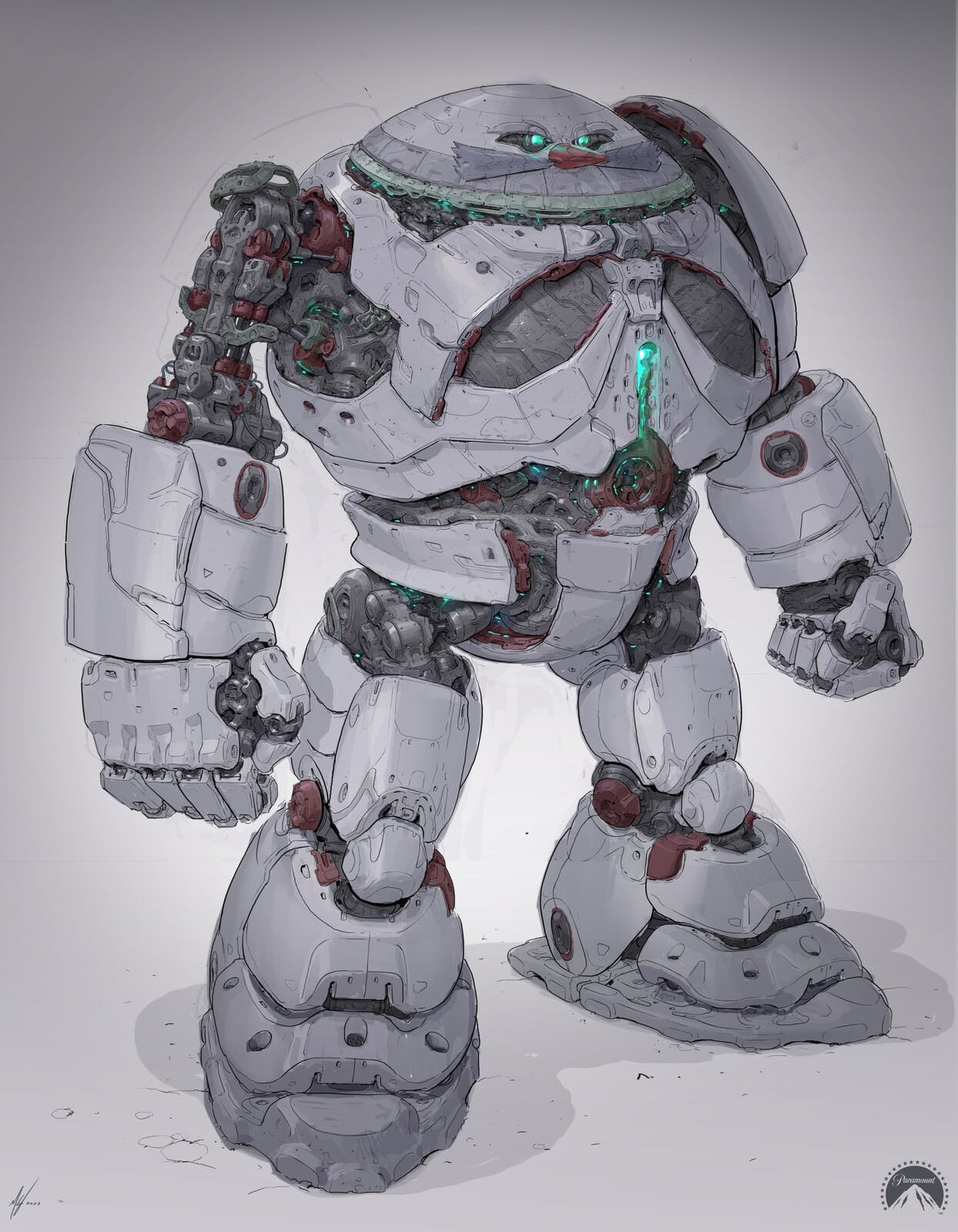The image showcases a concept art of a colossal gray robot, tall and dominating against a plain gray background. This robot exudes a mech-like presence with a dome-shaped, circular head featuring glowing green eyes, a pointy red nose resembling a cone, and a distinctive mustache and whiskers, reminiscent of Dr. Robotnik from the Sonic series. Its round body is predominantly light silver with darker silver leaf-shaped accents on both sides of the chest, converging towards a vertical green line that illuminates the center. The robot's thick and substantial arms are encased in robust gray armor, with the right upper arm partially exposed, displaying intricate mechanical details. Both legs are enormous, akin to cinder blocks, providing a sturdy and top-heavy appearance. The image is identified as concept art by a small Paramount Studios logo in the lower right corner and an artist's signature on the lower left.